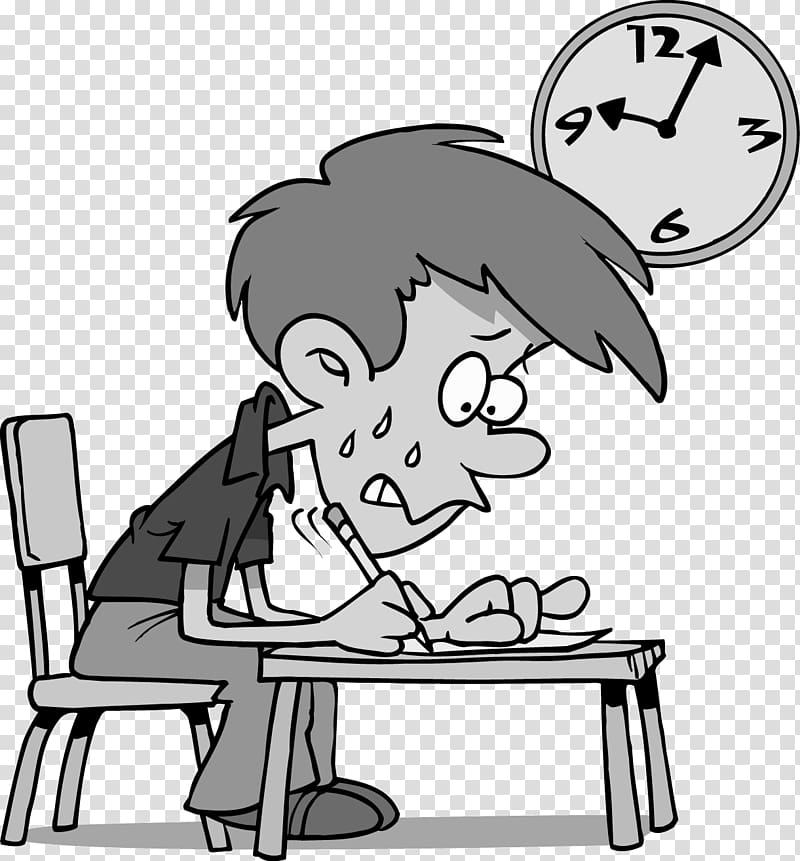The black-and-white illustration depicts a young boy or teenager sitting at a school desk, stressed out as he frantically writes on a piece of paper with a pencil. His hunched posture over the low desk suggests discomfort, and his facial expression, marked by a grimace with his lip biting and teeth showing, accentuates his anxiety. Sweat droplets are visible on his cheek, emphasizing his nervous state. He wears a collared short-sleeved shirt, long pants, and shoes. The background features a gray and white checkered pattern with a clock on the top right corner, indicating the time as slightly after 9 a.m. The boy's hair appears to be light in color, possibly light brown or red, and he has wide, panicked eyes with furrowed eyebrows, further conveying his stress as he writes furiously, illustrated by motion lines beside the pencil.